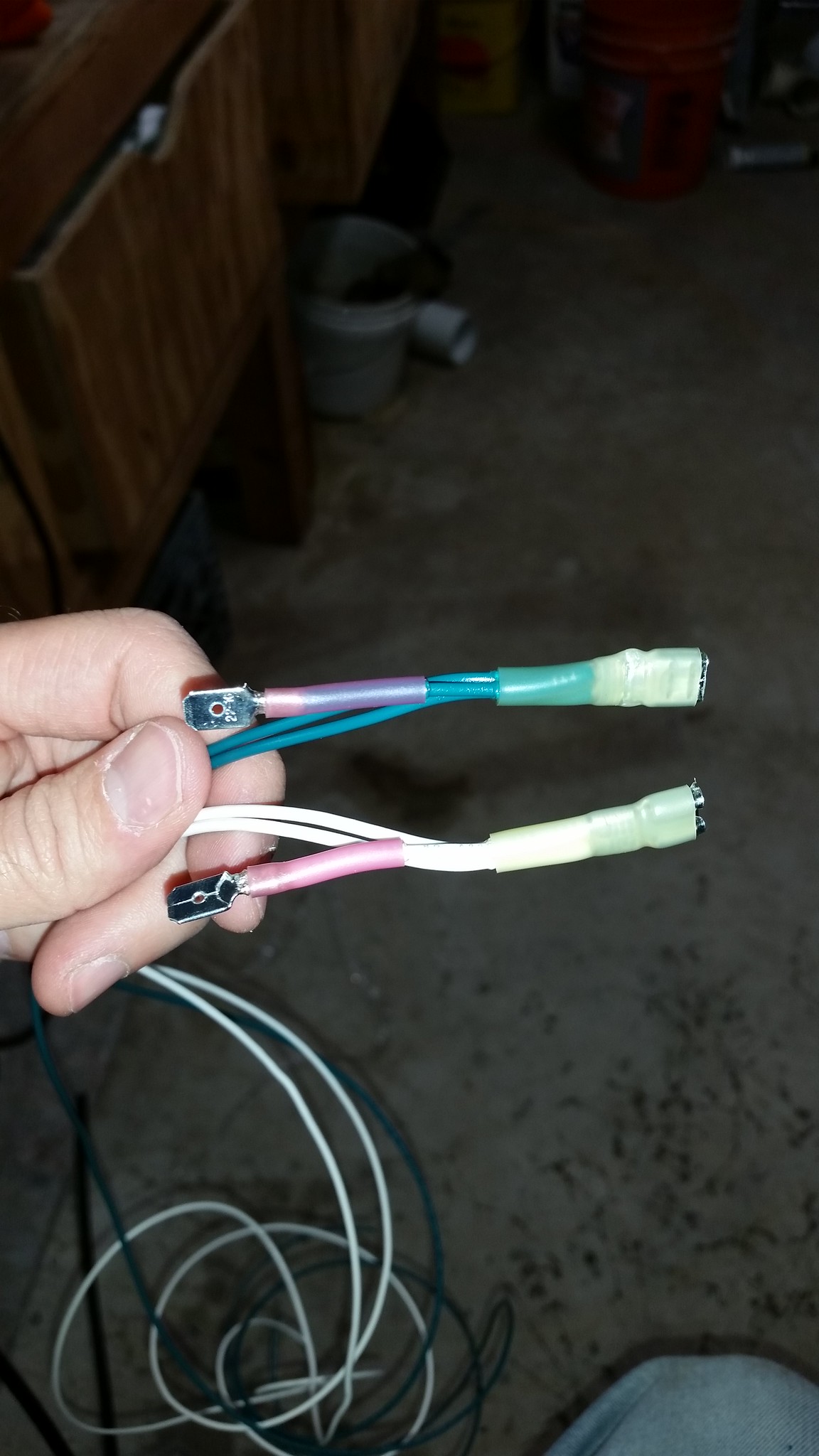The photograph showcases a dimly lit interior, likely a garage or workshop, characterized by a scuffed and dirty gray concrete floor. In the top-left corner, there is a dark brown desk accompanied by rough wood cabinets, and various buckets are scattered around; a gray one on the ground to the right, an orange one next to the top corner, and a red one in the center. A man wearing light blue jeans is partially visible, with only his knee in the frame. His Caucasian hand, with neatly trimmed nails, is extended from the left side of the image, holding two sets of cables.

The cables, which run horizontally across the middle of the photo, are prominently displayed. The top set consists of blue wires connected to an adapter piece wrapped in pink tape, with a small steel-colored tip. These wires appear to loop back towards another adapter piece and continue downward. The bottom set is similar, featuring white wires that follow the same looping pattern, also ending in adapters with pink sheaths and small metallic tips. The cables drape down and lie on the concrete floor, intertwining with each other.